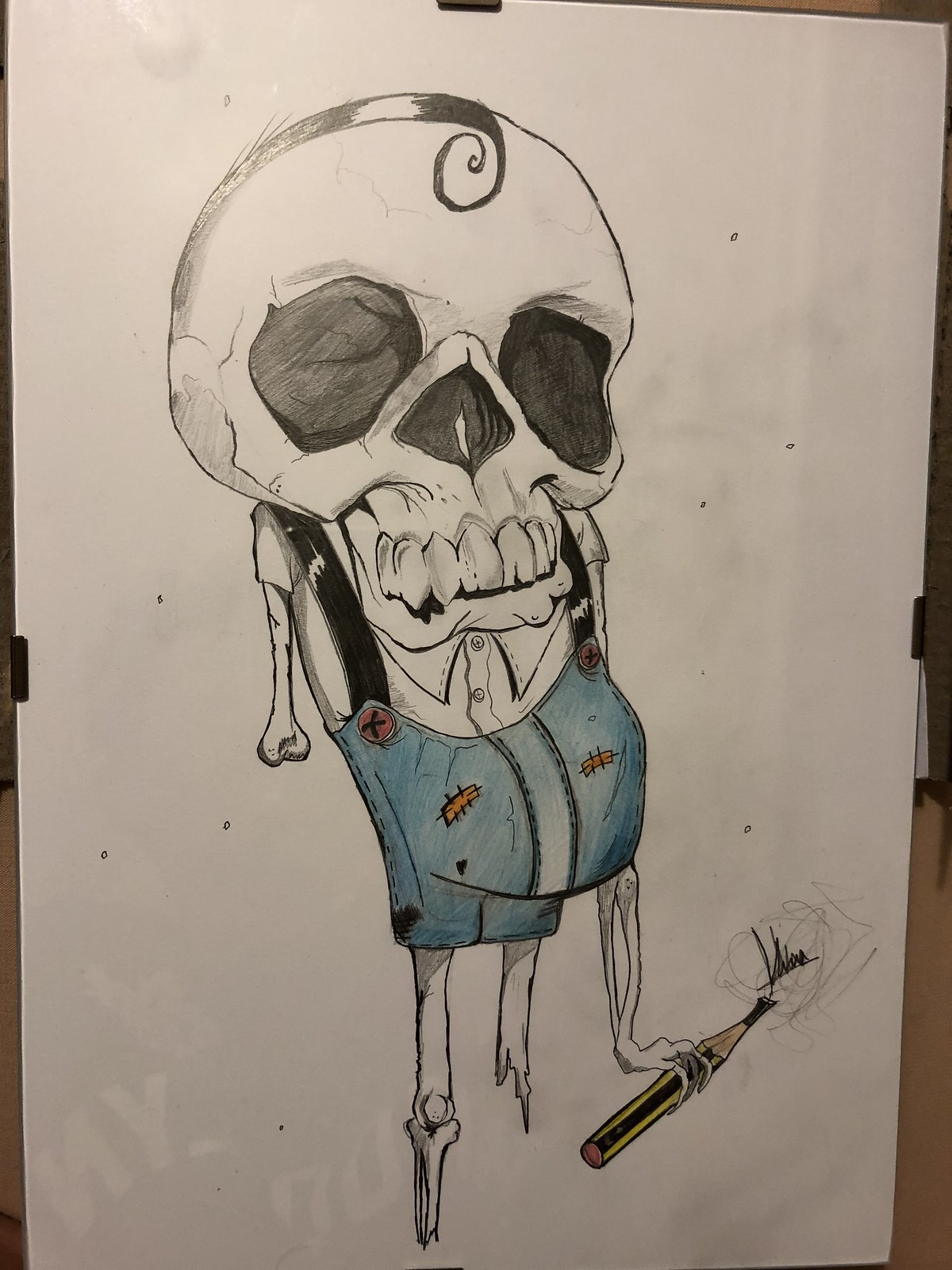This image features a meticulously detailed colored pencil drawing on a white page torn from a sketch pad, set atop a brown table-like background. The central figure of the drawing is a distinctive skeleton with a round skull and a narrow jaw, characterized by deep, empty eye and nose sockets. A notable feature is a tuft of black hair swirling in the center of the forehead. The skeleton's mouth, large and with a slight overbite, reveals an arrangement of visible teeth.

The skeleton is adorned in a short-sleeved, collared white shirt, which is complemented by black suspenders attached with brown buttons. The suspenders connect to blue overalls, worn and torn, adorned with brown patches, and forming a bulge at the stomach area. These overalls are quite short, stopping at the thighs, revealing partial skeletal legs, one side fragmenting just below the knee and the other stopping at the femur with a jagged end.

Remarkably, the skeleton’s left arm extends notably long, holding a yellow and black pencil with a pink eraser, seemingly writing the artist’s signature at the bottom left corner of the image. In contrast, the right arm comprises only a partial femur bone. The distinct placement and details, combined with the visual elements, reflect a creative and whimsical representation of skeletal life.